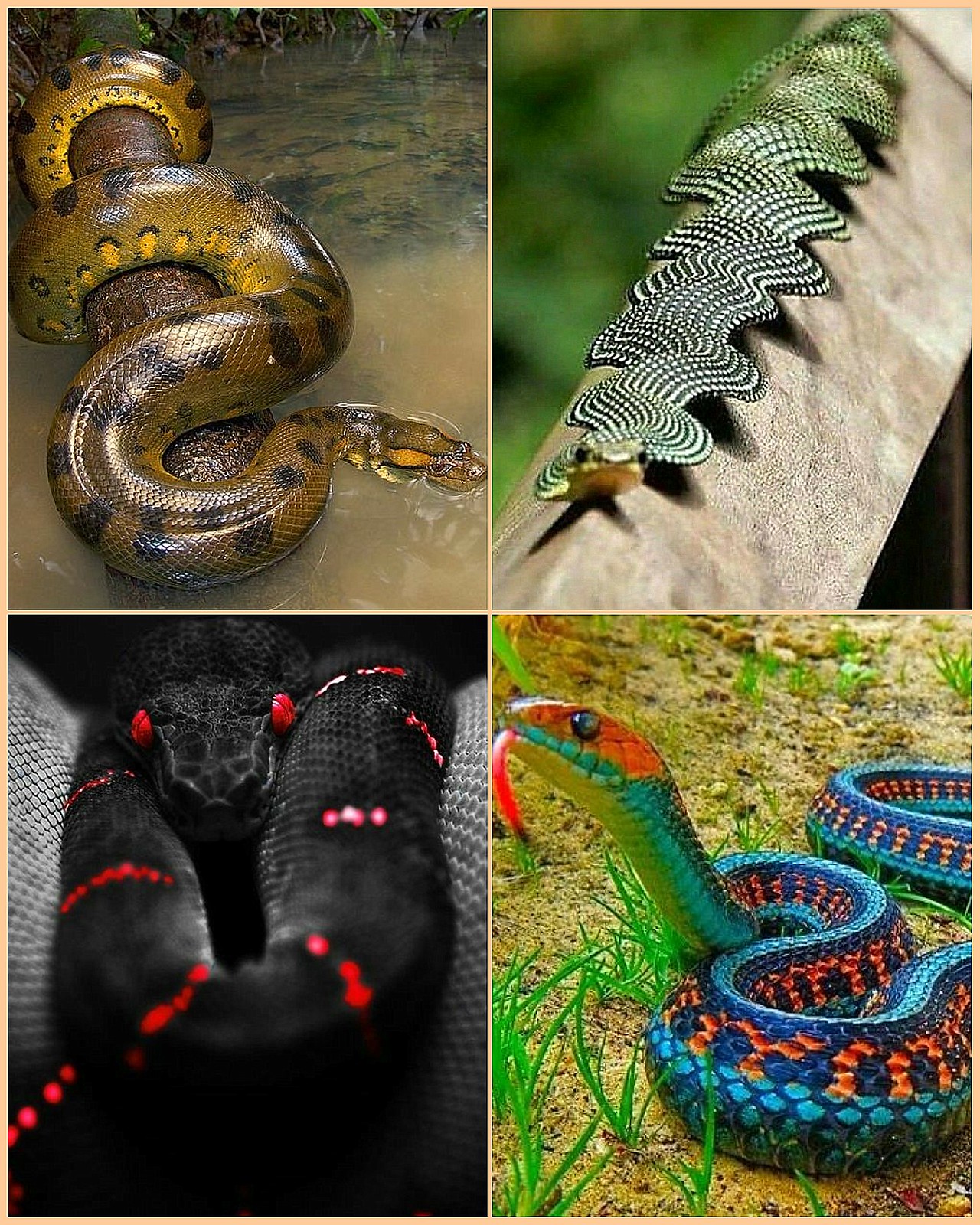This composite image showcases four distinctive snakes, each inhabiting unique environments. The upper left quadrant features a massive anaconda or python with a thick, brown body accentuated by black spots, wrapped intricately around a log within a swampy jungle setting. Moving to the upper right, there is a slender, leaf-like snake with a gold hue, adorned with white polka dots and a wavy pattern, positioned elegantly on a branch amidst a blurred vegetative background. On the bottom left, a menacing black snake with glowing red eyes and striking red stripes commands attention, possibly situated against a monochromatic scaly texture, contributing to its eerie allure. Finally, the bottom right segment presents a vivid, indigo-styled snake exhibiting a mosaic of baby blue, dark blue, and orange hues, eyes intent, and tongue out, as it slithers over a dry, cracked dirt terrain interspersed with sparse green shoots. While the authenticity of these serpents—whether real or AI creations—remains ambiguous, their striking designs and diverse habitats create a captivating visual narrative.